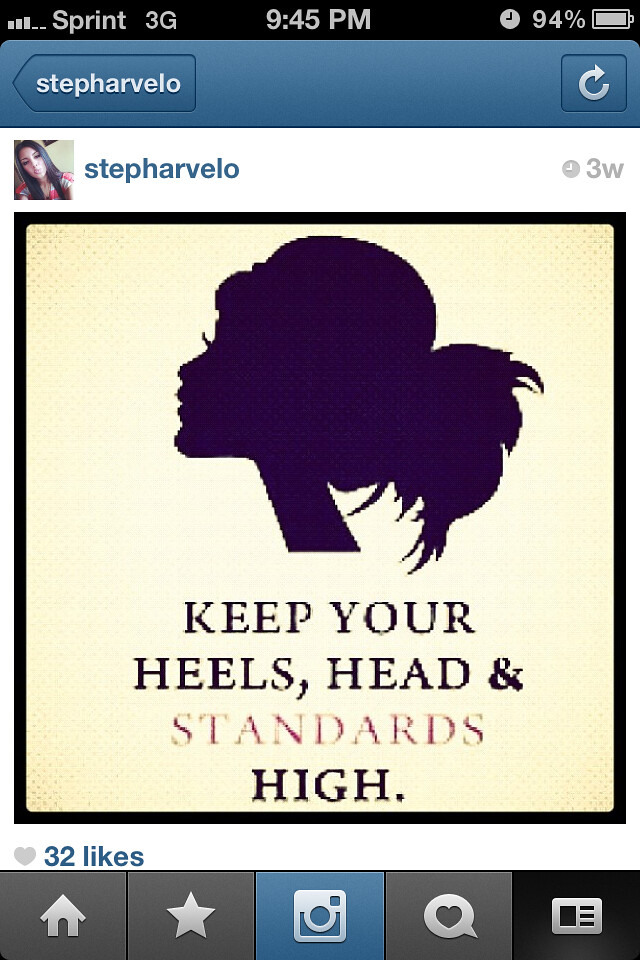This image displays a screenshot from a cell phone. It shows the status bar at the top with "Sprint 3G," a signal icon, "9:45 PM," and a 94% battery level on a black background. Below the status bar is a blue banner that spans the screen, displaying the name "STEP HARBELO" and a refresh button on the right. Directly below the blue banner is a white strip with a small picture of a woman with dark hair next to the name "STEP HARBELO" in blue text, followed by a small clock icon and "3w." The main section of the screen features a black silhouette of a woman with a large bun and a skinny neck against a purplish-black background, accompanied by the quote "Keep your heels, head, and standards high." At the bottom of this section, it shows "32 likes" alongside a row of icons typical for social media, including a heart, house, star, camera, and another symbol.